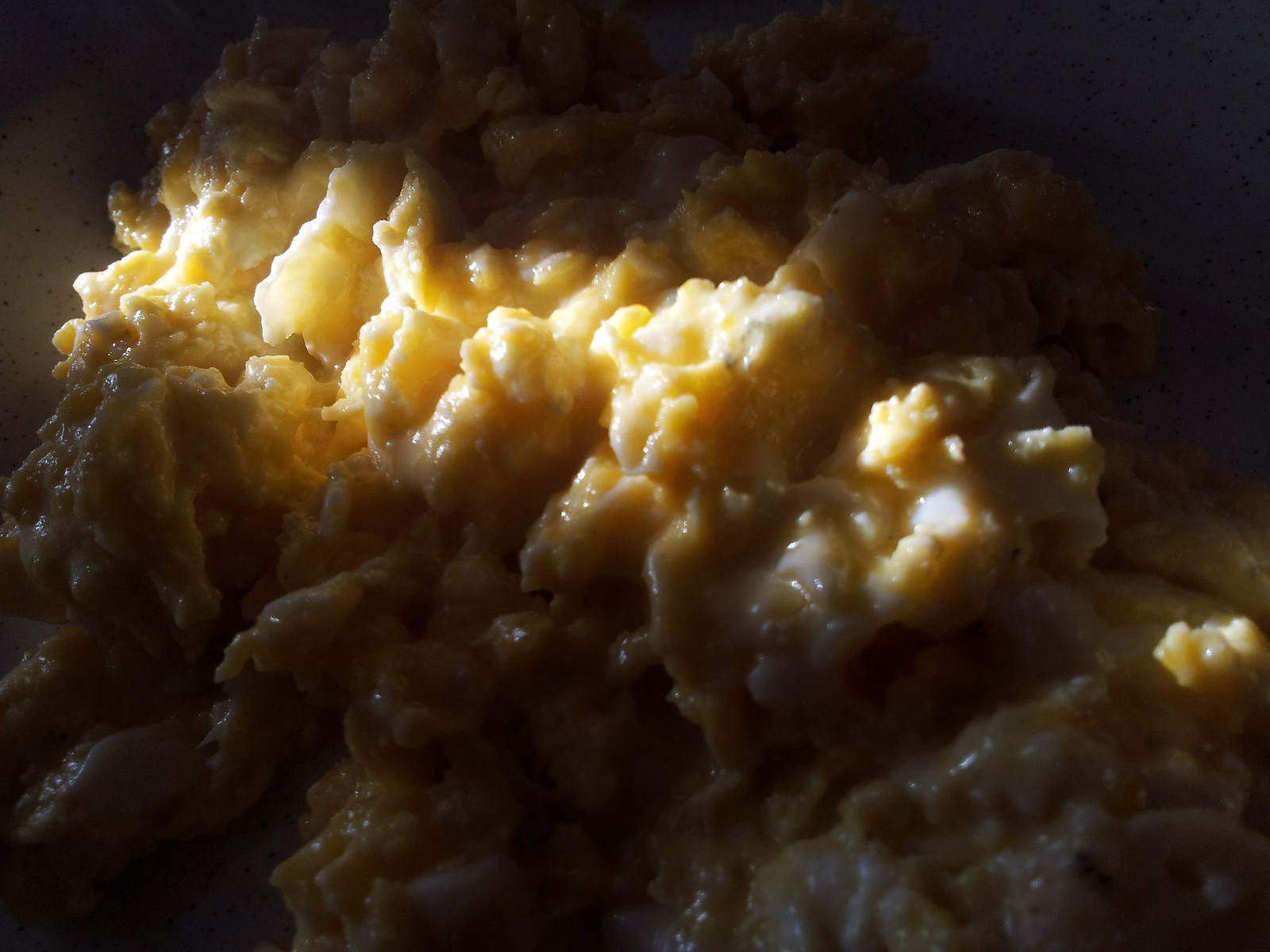In this color close-up image, we are presented with a perplexing scene, predominantly shrouded in shadow, with only a narrow strip of light illuminating a portion of the subject. The illuminated area reveals a lumpy, semi-solid mass that glistens, exhibiting a yellowish tinge. The mysterious substance is uneven in texture, featuring both solid and slightly gooey, liquid-like spots. The appearance suggests it could be a food item, with speculations ranging from scrambled eggs or cheese to a baked good like zucchini bread or banana bread, where the top surface has cracked and looks moist or gooey. The absence of text and the extreme zoom make it challenging to definitively identify the object, but the shared characteristics hint toward it being some form of yellow, semi-solid organic material, possibly a type of food prepared or in the process of being prepared.